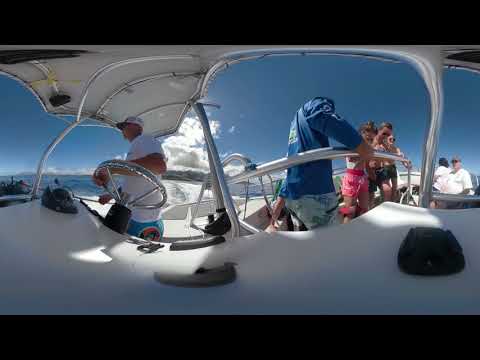In this vivid photograph of a sailing expedition, from left to right, the scene captures a lively group of people aboard a white sailboat with black, gray, and chrome trim, set against a backdrop of blue skies adorned with billowy cumulus clouds. On the left third of the image, a man with a white baseball cap, white short-sleeve shirt, and blue shorts stands at the chrome steering wheel, looking left. His left hand and forearm rest on the wheel, and he is shaded by the boat's covered awning. The boat portion where he stands is notably shady compared to the sunlit background.

Moving towards the right, the boat's uncovered section reveals more than five people, a mix of males and females. Among them, a male in a blue long-sleeve sweater and jeans stands out. Beside him, a woman sports pink shorts paired with a white shirt. Other individuals are casually dressed in white short-sleeve shirts and red or dark shorts. The photograph also offers a glimpse of the horizon and the water towards the left center, adding to the scenic maritime ambiance of the image.